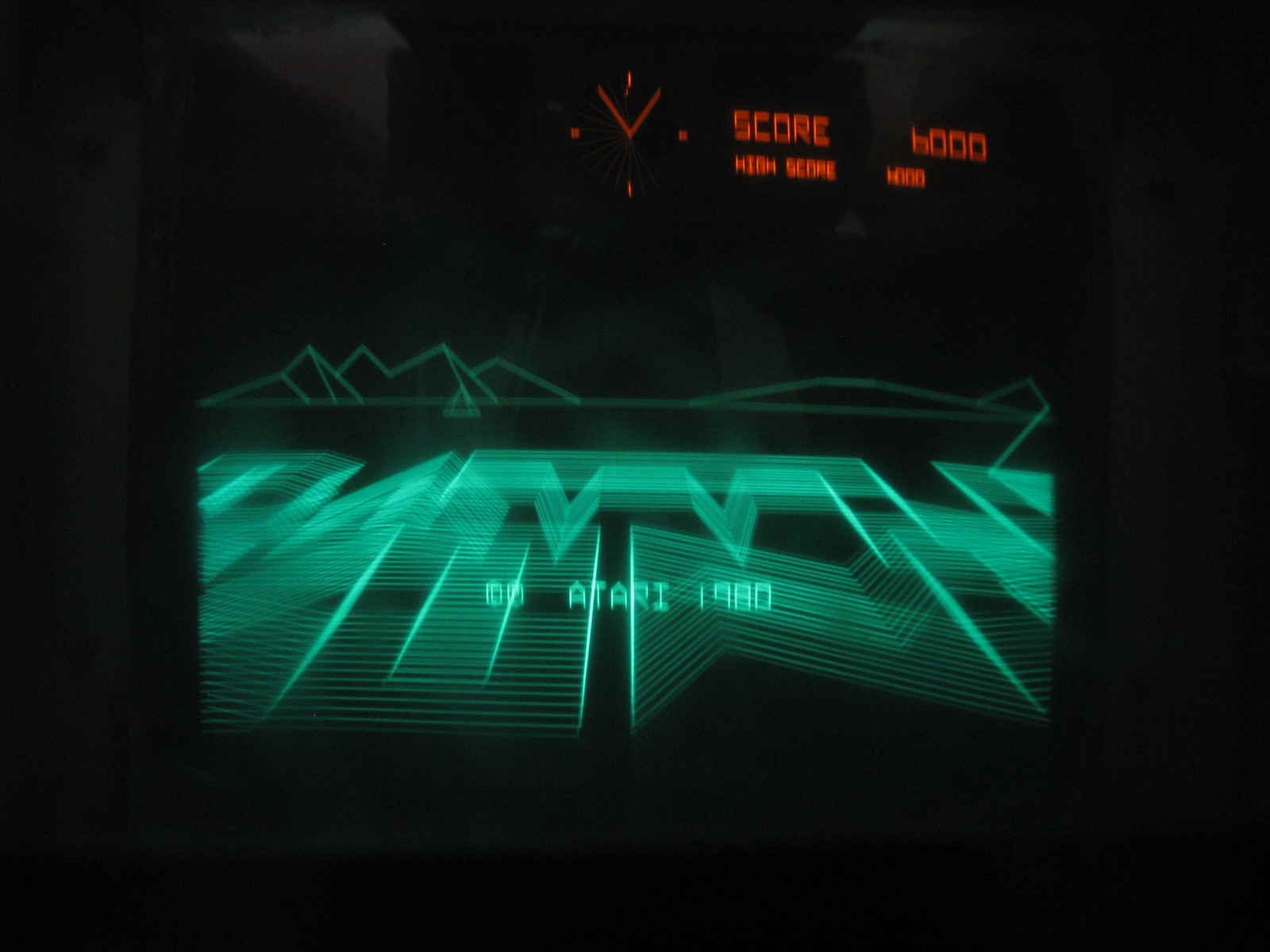The image depicts an Atari video game screen displayed on a television. The screen has a solid black background with various elements rendered in red. At the top of the screen, bold text reads "Score: 6,000" and "High Score: 6,000." Just to the left of this text, a red compass icon is visible. Below this, in the middle section of the screen, a graph-like design stretches horizontally, featuring thin lines that form a series of triangles and squares. At the bottom of the screen, a complex design composed of closely spaced thin stripes and asymmetrical shapes is present, adding to the intricate visual layout.